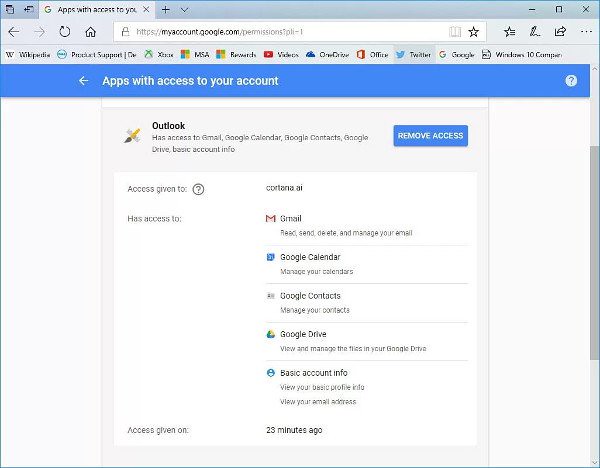The image is a screenshot captured from a computer screen displaying a browser tab open to the Google Account management page (myaccount.google.com). The top section of the page features a prominent blue banner reading "Apps with access to your account," followed by a white question mark icon. Below this banner, there is a specific entry indicating that Outlook has access to multiple components of the user's Google account, including Gmail, Google Calendar, Google Contacts, Google Drive, and basic account information. 

To the right of the list of services accessed by Outlook, a blue button labeled "Remove Access" in white letters is visible, suggesting that users can click it to revoke permissions. Additionally, the page notes that access was given 23 minutes ago. The detailed list highlights individual tabs related to Google Calendar, Contacts, and Drive under the access section.

At the very top of the browser, the user's assortment of favorite websites is visible, including icons for Wikipedia, Xbox, YouTube, and Twitter. The browser interface clearly shows this as a webpage the user has navigated to through a tab labeled "Apps with access to your account."